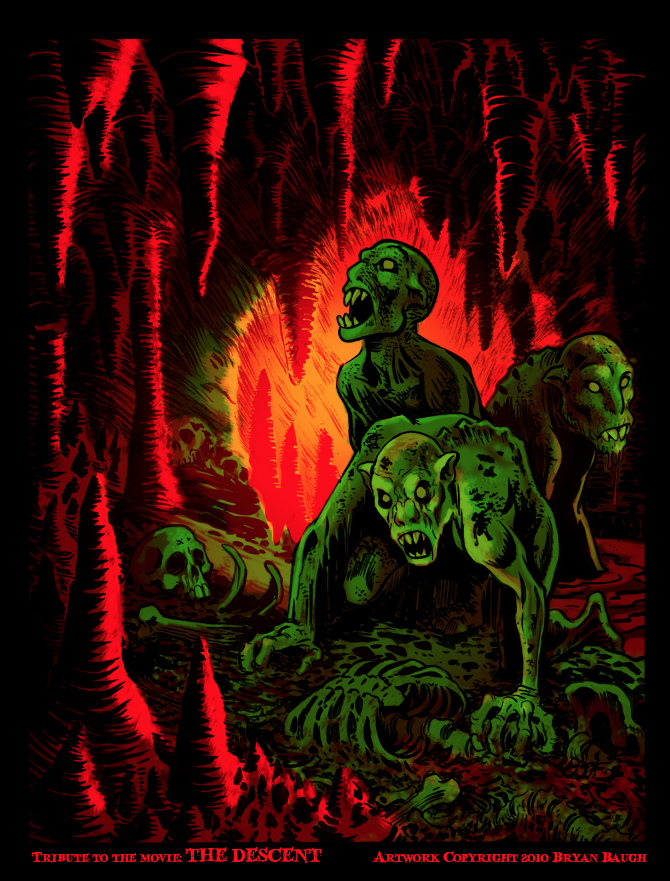This vividly detailed and intense graphic poster, created in 2010 by artist Brian Bach, is a tribute to the movie "The Descent." Set inside a glowing red and yellow cave, the artwork depicts three menacing, green, demon-like creatures crawling over skeletal remains including skulls and rib cages. The cave is adorned with sharp, pointy stalactites hanging from the ceiling and stalagmites pointing upwards from the floor, enhancing the ominous atmosphere. The creatures display a range of terrifying postures: one is down on all fours, while another leans forward with a menacing expression, and a third lifts its head to the sky, appearing to scream. Their mouths are filled with sharp teeth and sharp clawed hands add to their fearsome appearance. The dark, almost black background contrasts starkly with the bright, booming reds that light up the cave, creating an overall visually captivating scene that captures the essence of horror and dread. The lower corners of the poster feature text that marks the artwork as a tribute to the movie and credits the artist, Brian Bach.